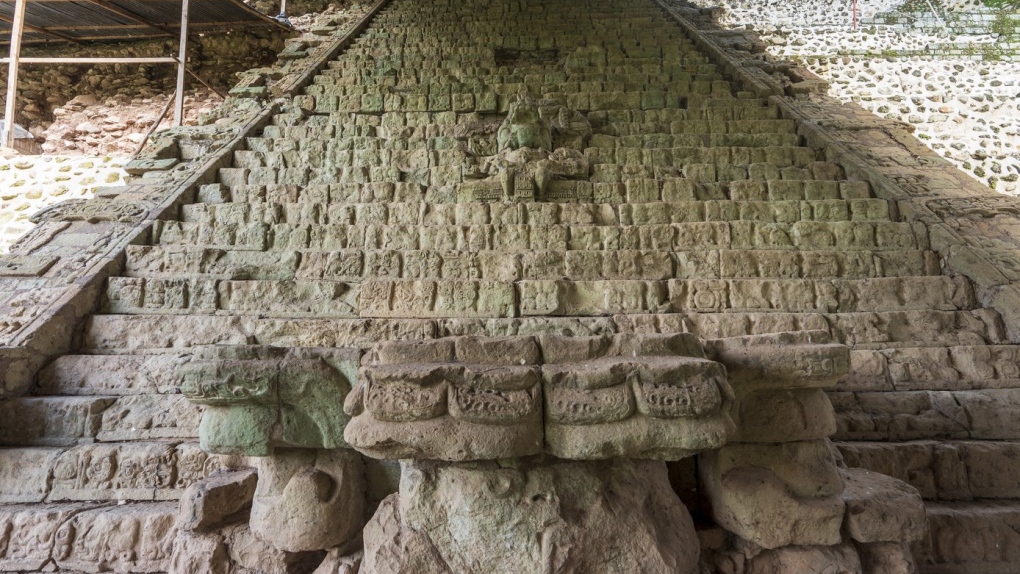The horizontal-rectangular image depicts the close-up front of an ancient and weathered stone building, partially in shadow. Decorative stone elements embellish the edges of the roof, while statues, likely depicting faded, unidentifiable figures, adorn the façade. The roofline extends above with additional stone structures visible in the background and alongside the building. Prominently featured in the foreground is a steep, old stone staircase, lined with intricate yet time-worn carvings. At the bottom of the staircase, two stone Chinese lions with expressive eyes and prominent manes sit majestically, flanked by indistinct, ancient animal figures. The stone steps ascend upwards, seemingly endless, bordered by inscribed white stone held together with clay, suggesting distinct Chinese architectural influences. The image, capturing the convergence of natural decay and historical artistry, gives a sense of an enduring pathway through a culturally significant location.